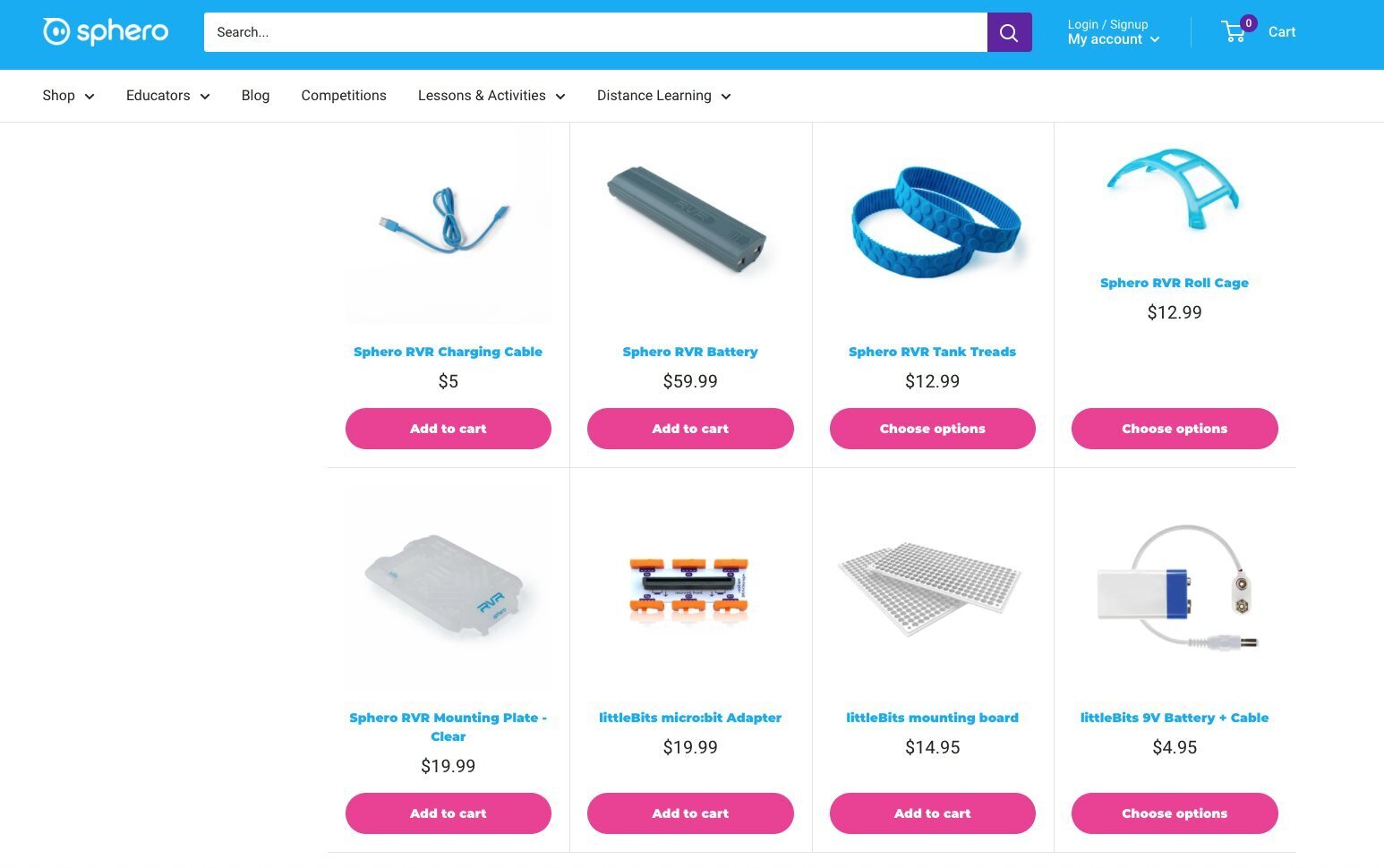On the webpage for Sphero, a company specializing in various tech items, the top of the screen features a prominent blue bar with the Sphero logo displayed in lowercase. Adjacent to the logo is a large, white search bar accompanied by a purple search icon. To the right, icons for logging into accounts and viewing the shopping cart are present, with the latter indicating zero items.

Below the blue bar, there are several dropdown menus labeled: Shop, Educators, Blog, Competitions, Lessons and Activities, and Distance Learning, suggesting a strong focus on educational technology.

The main body of the page showcases an array of Sphero accessories arranged in a 4x2 grid format. Each item is accompanied by a small image and brief description. The first row includes:

1. Sphero RVR Charging Cable - Priced at $5, with an option to add to cart.
2. Sphero RVR Battery - An accessory for an unspecified Sphero tech device.
3. Sphero RVR Tank Treads - Likely suggesting the device is some type of electric vehicle, priced at $12.99.
4. Sphero RVR Roll Cage - Indicating the device might be a motorized toy, like a small vehicle.

The second row features:

5. Sphero RVR Mounting Plate - Available for $19.99.
6. LittleBits Micro USB Adapter - Priced at $19.99.
7. LittleBits Mounting Board - Available for $14.95.
8. LittleBits Nine Volt Battery + Cable - Priced at $9.00.

The descriptions suggest this page is designed to order various accessories for a tech device known as Sphero RVR, which appears to be an educational technology tool likely involving a small robotic vehicle.